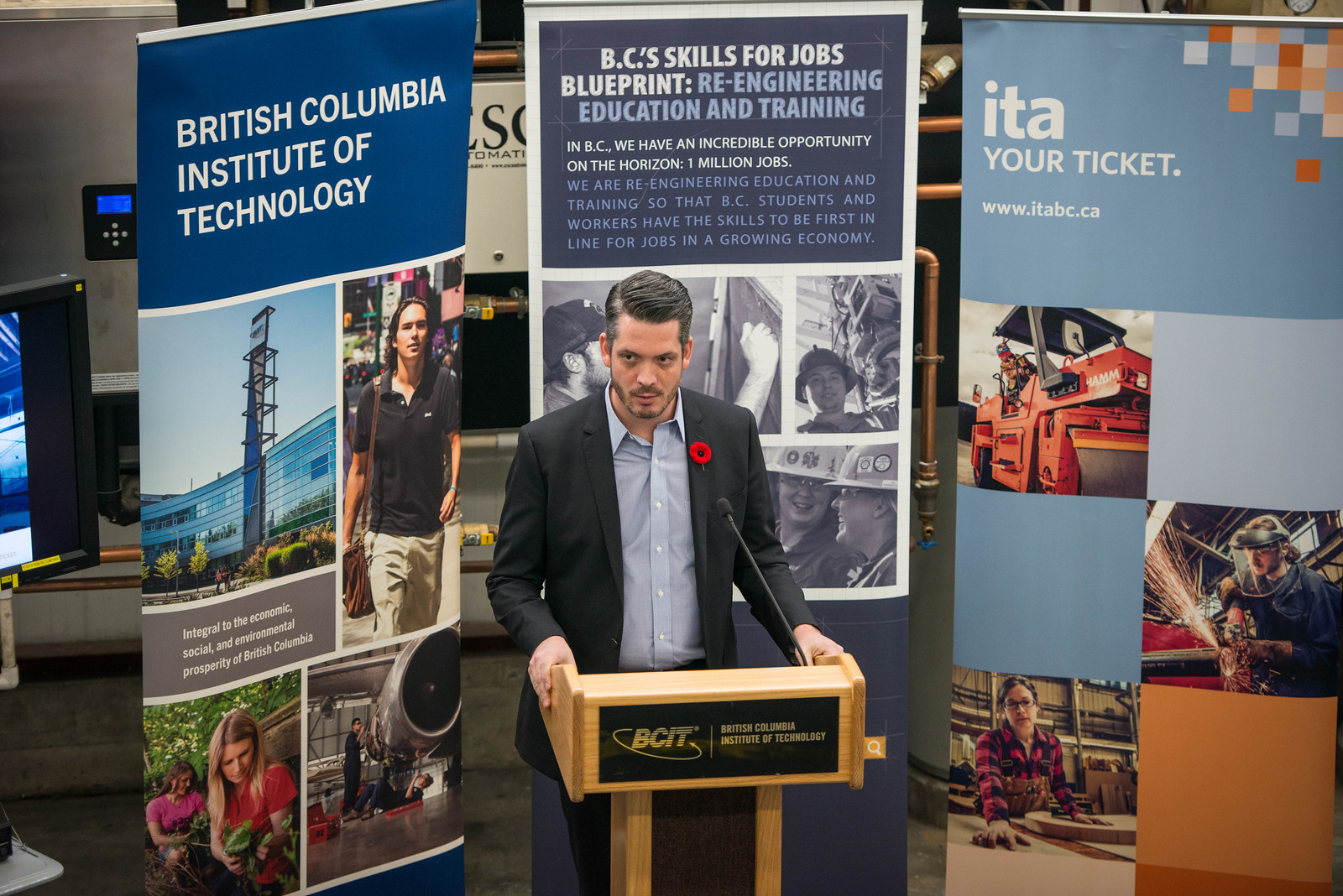In the image, a man stands as the focal point behind a light wooden podium. The podium features a black panel with gold text that reads "BCIT, British Columbia Institute of Technology," and has a microphone extending from its top. The man has dark, side-combed hair, a mustache, and a bit of a beard. He is dressed in a dark gray suit jacket over a blue collared button-up shirt, adorned with a red flower pinned to his lapel. Behind him, three blue-themed banners showcase various scenes: a welder, a woman tending plants, and additional imagery of people engaged in different activities. These banners also carry text such as "British Columbia Institute of Technology," "BC Skills for Jobs Blueprint: Re-engineering Education and Training in BC," and a promotional message about job opportunities and training. Visible through the gaps between the banners, the rest of the room contains miscellaneous items like brass pipes, a computer monitor, and additional signs.